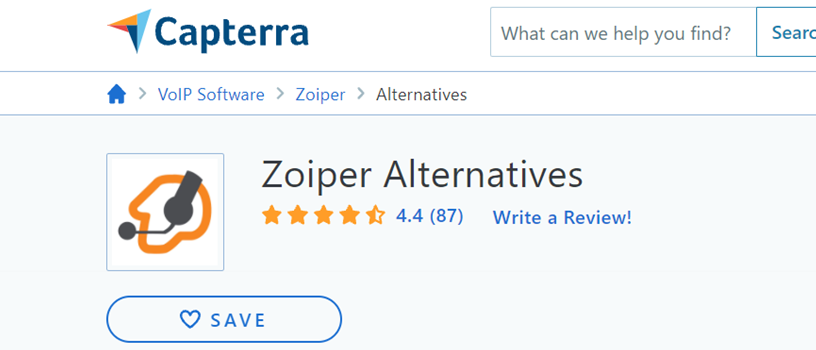This is an image of the website Capterra. At the top, the Capterra logo features an arrow pointing to the northeast, with a gradient comprising light blue, dark blue, red, and orange colors. To the right of the logo, there's a search bar with the prompt, "What can we help you find?" 

Below the header, a breadcrumb navigation trail is visible. On the far left is a house icon representing the home page, followed by an arrow pointing to "VOIP software," another arrow leading to "Zoiper," and yet another arrow pointing to "alternatives." 

Beneath the breadcrumbs, there is an icon of a person wearing a headset next to the text "Zoiper Alternatives." Below this header, the rating section displays a 4.4 out of 5-star rating, based on 87 reviews. 

To the right of the reviews, there is a blue button labeled "Write a Review!" Further down, another button that says "Save" features a blue outline and a blue heart symbol inside it. 

The overall design of the website is white and clean, providing a clear layout and easy navigation.